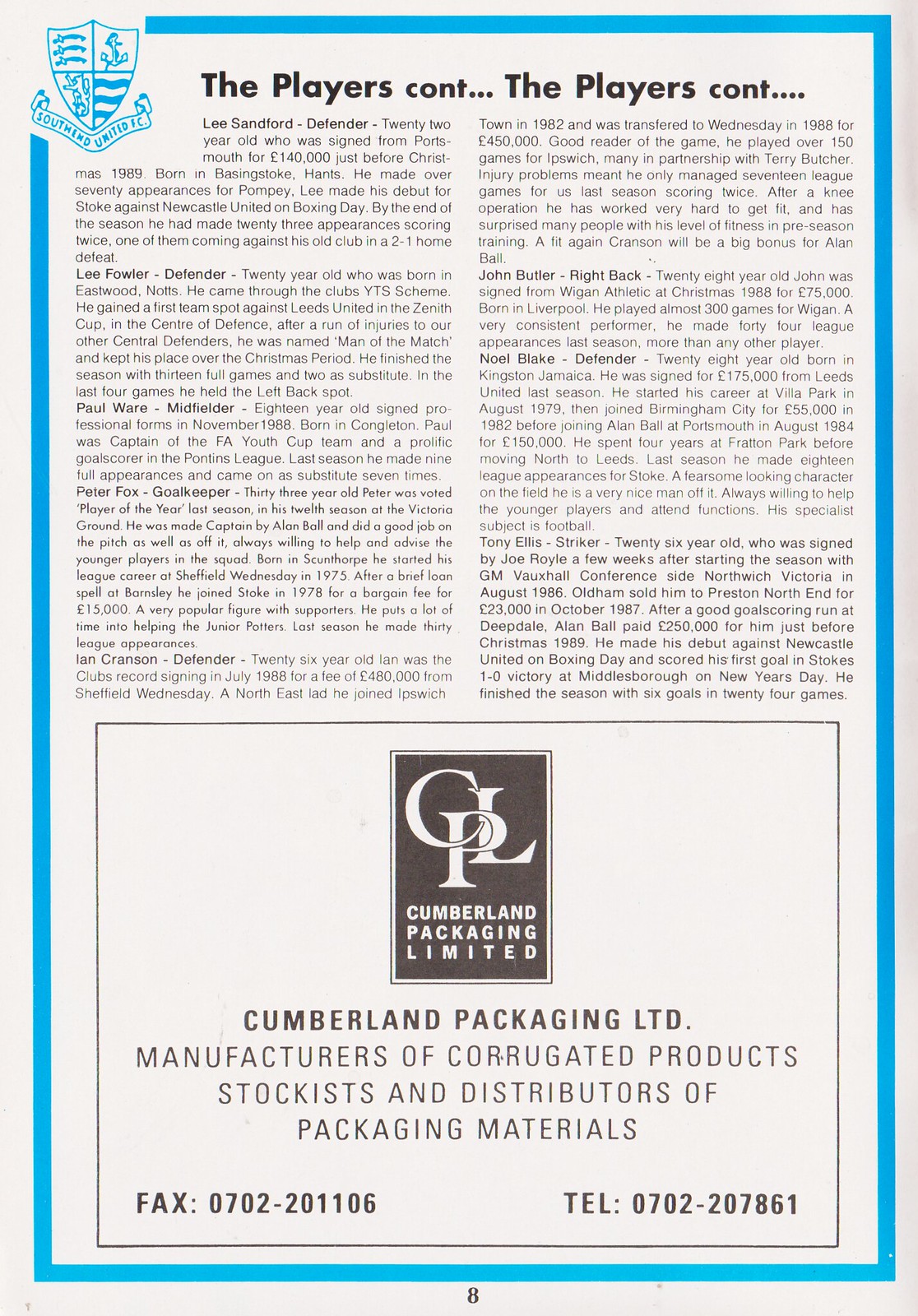This is an image of page eight from a sports program or catalog, featuring a white background with a light blue border running all the way around except at the top, where there is a blue shield emblem for Southland United with various symbols and an unreadable banner beneath it. The page's header reads, "The Players Continued..." and is organized into two newspaper-style text columns. Each column contains bolded names and paragraphs of text detailing player profiles. The left column starts with Lee Sanford, a 22-year-old defender, followed by Lee Fowler, another defender, and Paul Weard, a midfielder. Peter Fox, a goalkeeper who has the longest biography, is also included. The right column features players such as John Butler, a right back, an old Blake defender, and Tony Ellis, a striker. The bottom 40% of the page is dedicated to an advertisement for Cumberland Packaging Limited. The ad features a rectangular blue logo with the letters CPL and text stating the company is a manufacturer of corrugated products and a distributor of packaging materials, with their fax and telephone numbers provided. The page number "8" is centered at the very bottom.